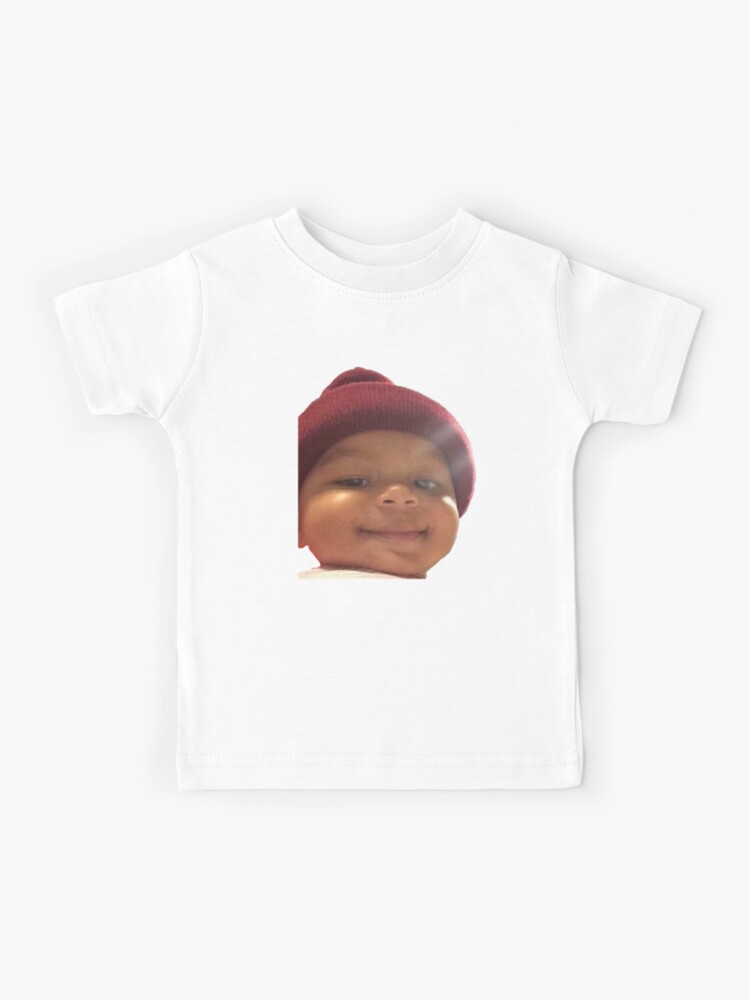The image features a plain white, crew neck t-shirt hanging against a white background. The t-shirt displays a photorealistic, silkscreen print of an adorable baby with light brown skin, a wide, closed-mouth smile, and chubby cheeks, suggesting that the child is around one year old. The baby, who could be African-American or possibly of mixed race, is wearing a maroon-colored beanie with a pom-pom on top. His bright, expressive brown eyes and joyful expression add warmth to the image. Notably, the left side of the baby’s head in the print is cut off at a straight edge, giving it an amateurish feel. Overall, the t-shirt exudes a handmade charm despite its imperfections.